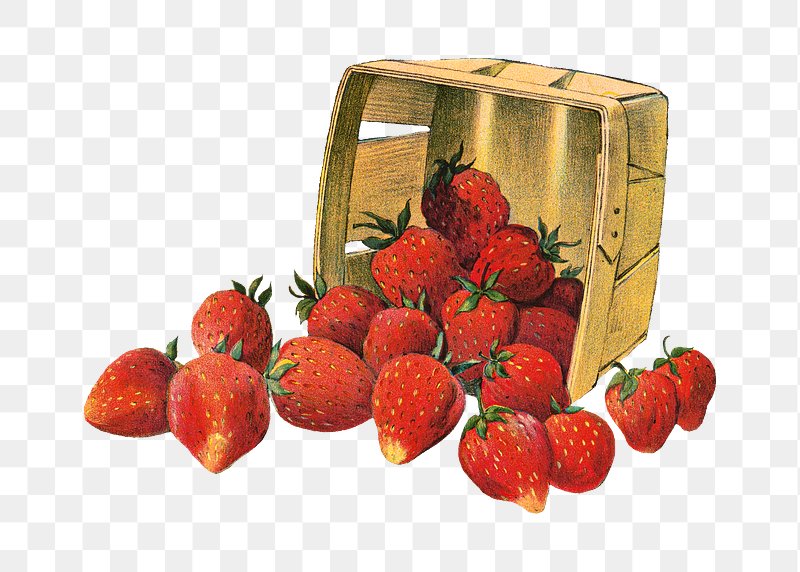This detailed cartoon illustration features a wicker basket intricately drawn in light brown/tannish hues, turned on its side, spilling vibrant red strawberries. Set against a transparent background depicted with a checkered white and grey pattern, the vividly colored strawberries, characterized by their yellowish seeds and green stems, scatter across the foreground. The strawberries inside the basket, which showcase detailed shadowing towards the back, hint at the meticulous effort put into the artwork. A few strawberries remain inside the square basket, while the majority tumble out, some towards the forefront and others to the right side of the image. There are neither additional objects nor figures, keeping full focus on the realistically portrayed fruit and basket.